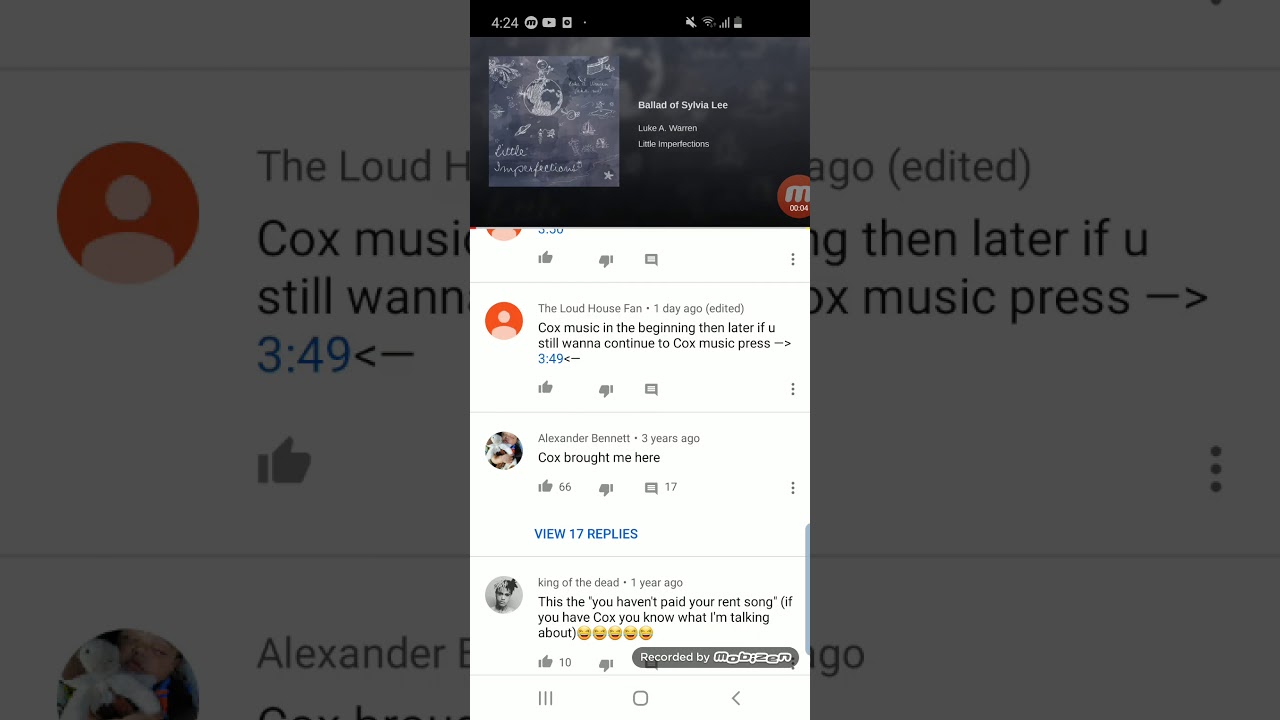In this composite image, two distinct sections are presented. The first section features a small rectangular image centered on the top half of the main image. It is characterized by a black background at the top, with white text "424" prominently displayed. Surrounding this, there are white icons indicating Wi-Fi signal strength and a low battery status. The middle of this section transitions into a grayish background, interrupted by an orange circle containing a gray 'M'. Below this, the section appears to show a digitally altered off-white photograph against a gray backdrop.

The lower section of the main image contains a comment thread. The background is predominantly white. It starts with a comment from a user named "The Loud House Fan", posted one day ago. The user's profile icon is a red circle with an image of a person’s face. The comment, partially unedited and edited, mentions Koch music repeatedly. For emphasis, certain text such as "3-49" is highlighted in blue. Below this, social interaction icons for likes, dislikes, comments, and more options are displayed.

Following this, another user, Alexander Bennett, comments three years ago indicating, "Kochs brought me here," followed by the same interaction options and an additional link in blue to "view 17 replies".

Further down, a comment from "King of the Dead" posted one year ago references a song humorously dubbed "you haven't paid your rent song", accompanied by laughing face emojis. Similar interaction icons and a gray circle indicating the track being "recorded by" are included here. The background of this lower section includes a superimposed image referring back to the comment from "The Lord House Fan".

Overall, the composite image juxtaposes varying degrees of content, including user comments, icons, and digitally altered elements, all set against a contrasting background palette.